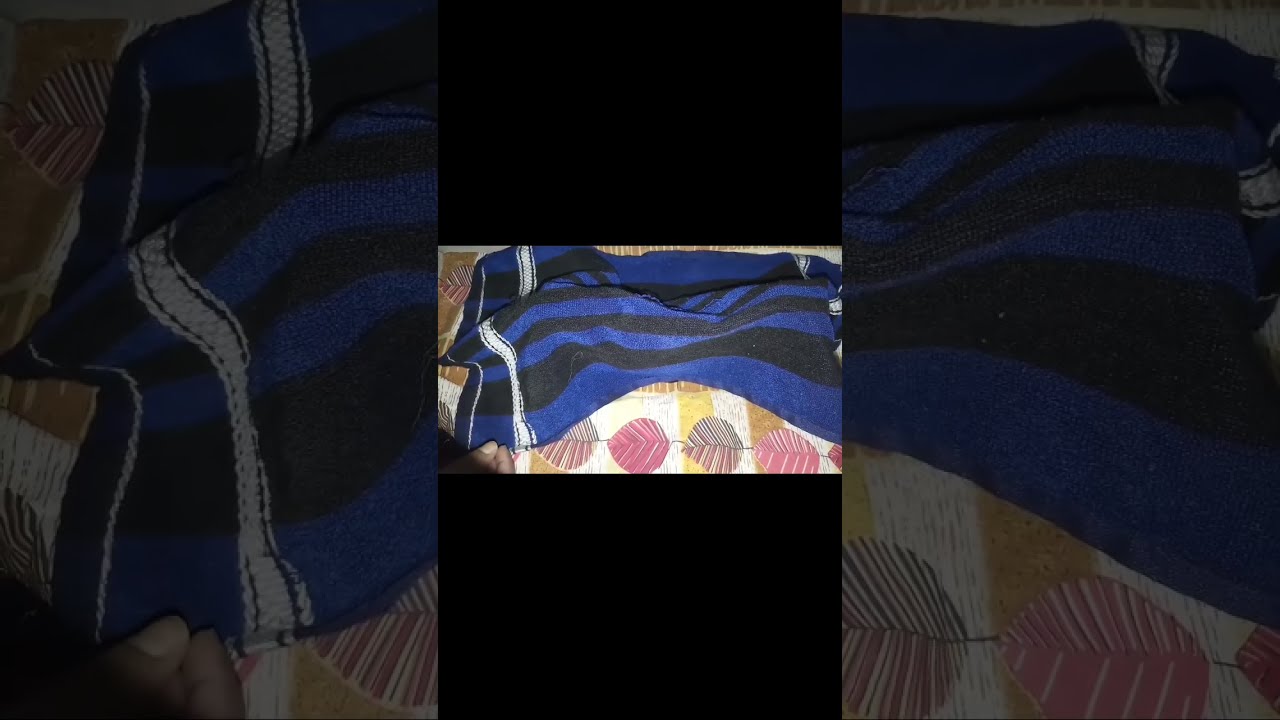The image features a detailed and vibrant centered composition framed by extensive black sections at the top and bottom, occupying a third of the picture each. In the center, a clear, color image showcases two blankets layered one over the other. The upper blanket is striped in blue and black with two additional vertical white stripes on the far left and right, one thick and one thin. This blanket is held at the corner by a hand. Beneath it lies a second blanket adorned with a pattern of leaves and stripes in various shades of mauve, brown, red, white, and yellow. The clarity and richness of the colors make the details stand out prominently against the black background.